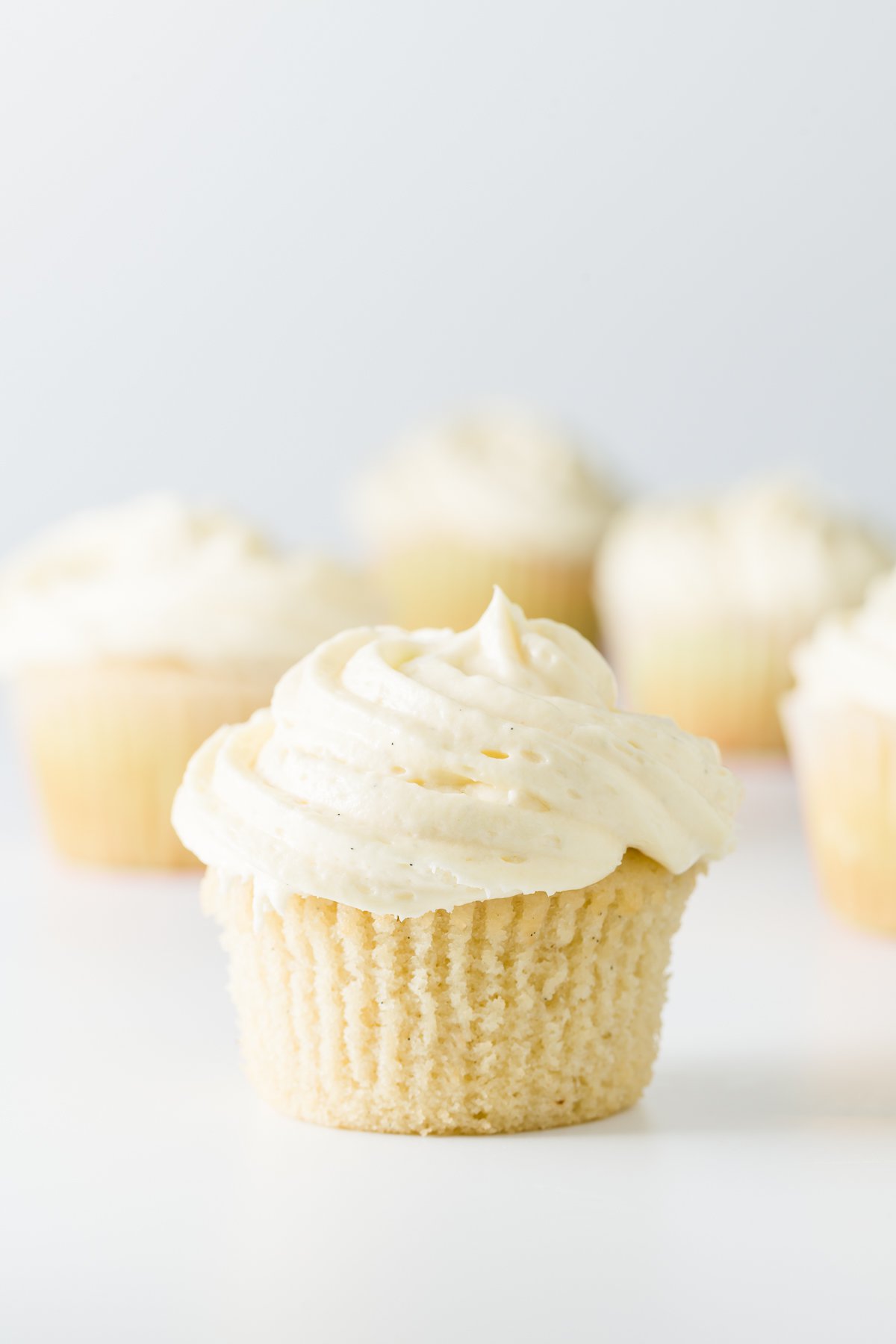A close-up side view of a freshly baked tan cupcake with white, whipped cream-like frosting serves as the focal point in this bright, indoor photograph. The large, unwrapped cupcake at the center prominently displays the horizontal ridges from its former paper liner. The frosting swirls elegantly atop, peaking slightly in the middle. Set against a light blue background, the cupcake sits on a shiny, white marble table. Slightly out of focus in the background, four additional cupcakes, identical in appearance, line up from left to right, subtly hinting at a series. The absence of any text or wording further emphasizes the image's intent to highlight the cupcake's appealing presentation, likely for advertisement purposes.